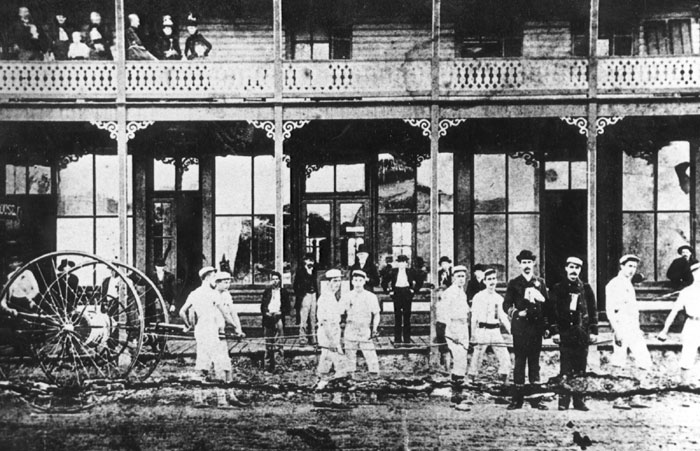This black-and-white photograph, likely from the late 1800s or early 1900s, depicts a street scene in front of a large, ornate two-story building that resembles a hotel. The building features several large windows and French doors, with a balcony on the second floor that has detailed railings. On the balcony, a group of people, both men and women, dressed in period attire with hats, are gathered towards the upper left corner, observing the scene below.

In the foreground, a group of predominantly young men are dressed in light-colored uniforms and white newsboy caps. They appear to be pulling a large, wheeled apparatus that has two oversized iron wheels and poles extending out from it, possibly a cart or an elaborate piece of equipment. The ground they're standing on looks muddy and wet, indicating poor weather conditions.

To the far right of the image, two well-dressed men in dark suits and hats stand facing the camera, possibly overseeing the activity. This dynamic image captures a moment in time, bustling with life and activity, yet steeped in the historical aura of its era.